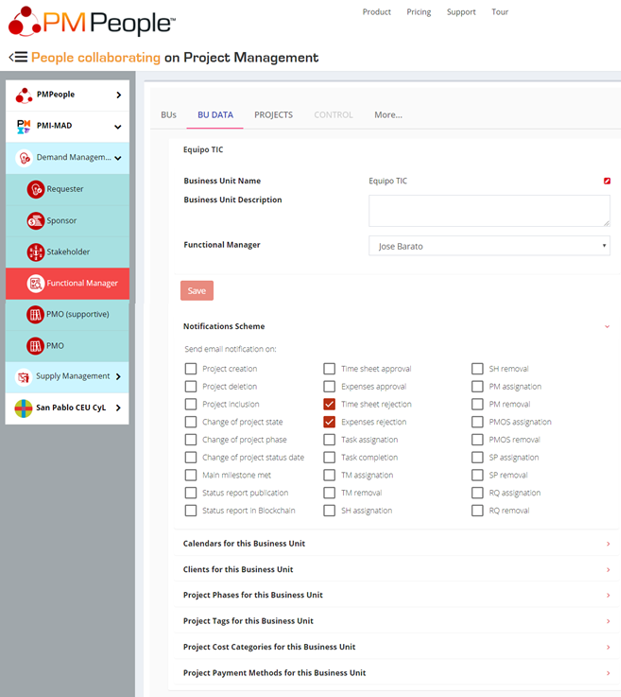This image represents a detailed screen capture from a project management website interface. At the top-left corner, there is a distinctive red icon comprising three concentric red circles. Adjacent to this, in orange text, is the label "PM" (likely indicating Project Management), followed by the black text "people". Additionally, an orange icon depicting collaboration is visible, alongside the black text "on product management".

The left sidebar is white against a gray background and features various white boxes with black font text labels. This area hosts a series of colorful icons in red, black, orange, purple, and blue, each representing different roles and functions within the project management system. These icons are labeled as follows: PM people, PMI MAD, demand management, requester, sponsor, stakeholder, functional manager, PMO supportive, PMO, supply management, and San Pablo CEU.

On the right side of the screen, against a white background, several categories are organized for ease of navigation. These categories are headed as BU's (Business Units), BU data, projects, control, and more. The "BU data" category features navy font with a pink underline and includes fields designated for “business unit name” and “business unit description” in black font, complemented by white text boxes. This section also includes drop-down menus for selecting a functional manager.

A prominent red "Save" button is visible for saving data entries. Below it, in black text, is the "notification scheme" heading, followed by a series of white and gray boxes with gray font labels for various notifications. The ticked items in red and white are "timesheet rejection" and "expenses rejection".

Further down, a gray section addresses various aspects of business unit management, with headings such as "calendars for this business unit", "clients for this business unit", "project phases for this business unit", "project tags for this business unit", "project cost categories for this business unit", and "project payment methods for this business unit".

Overall, this screen capture illustrates a comprehensive project management tool interface with detailed functionalities for managing business units, notifications, and project-related elements.